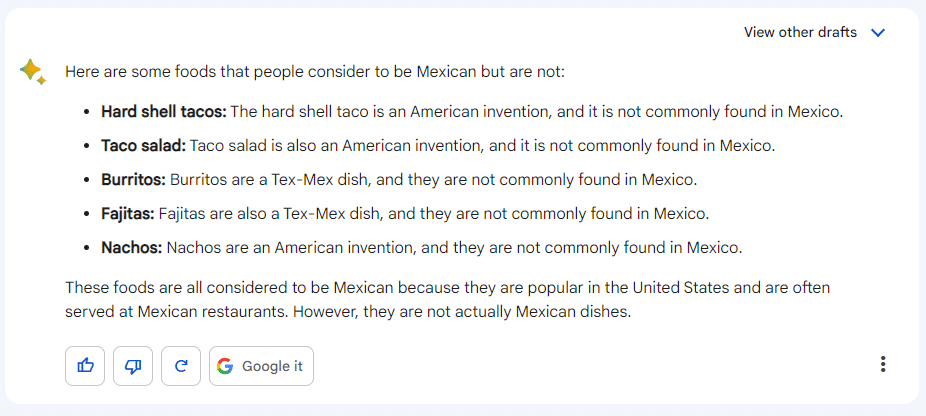This screenshot appears to capture content from a computer screen, as suggested by its wide, elongated dimensions typical of a monitor. In the upper right-hand corner, the text "View Other Drafts" is displayed in black font, accompanied by a blue downward-pointing arrow. On the left side, a cluster of decorative stars in yellow, blue, red, and green adorns the image. Adjacent to these stars, a heading reads: "Here are some foods that people consider to be Mexican but are not." 

Beneath this heading, there is a list of five bullet points in bold text:

1. Hard shell tacos
2. Taco salad
3. Burritos
4. Fajitas
5. Nachos

Additional explanatory text clarifies that:
- Hard shell tacos are an American invention and not commonly found in Mexico.
- Taco salad is also an American creation and is rarely seen in Mexico.
- The remaining items, burritos, fajitas, and nachos, similarly do not originate from traditional Mexican cuisine.

This detailed layout outlines common misconceptions about certain foods and their origins.